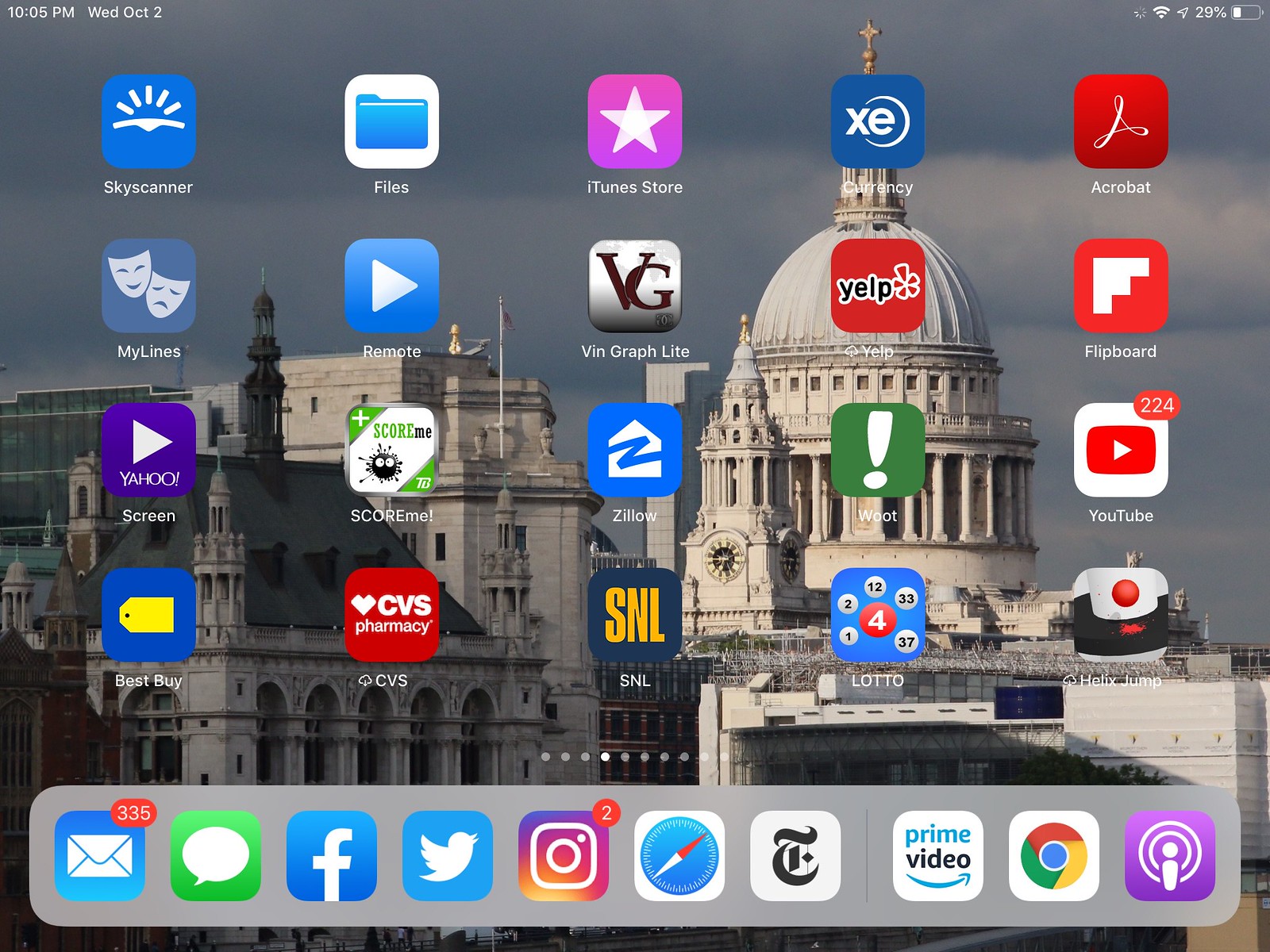This image is a screenshot taken from a computer screen, showcasing a total of 30 icons. The icons are arranged with 25 icons visible on the main part of the screen and an additional 10 icons along the bottom. Prominent among these are icons for CBS, Best Buy, "Saturday Night Live" (SNL), Zillow, Yelp, iTunes, Adobe Acrobat, Flipboard, YouTube, Amazon Prime Video, The New York Times, Facebook, MyLines, Skyscanner, a file manager, and a lottery application. The background features a scenic architectural photograph, depicting an old-fashioned building under a clear blue sky dotted with white clouds. The mix of application icons alongside the vintage architecture creates a contrast between modern technology and timeless design.